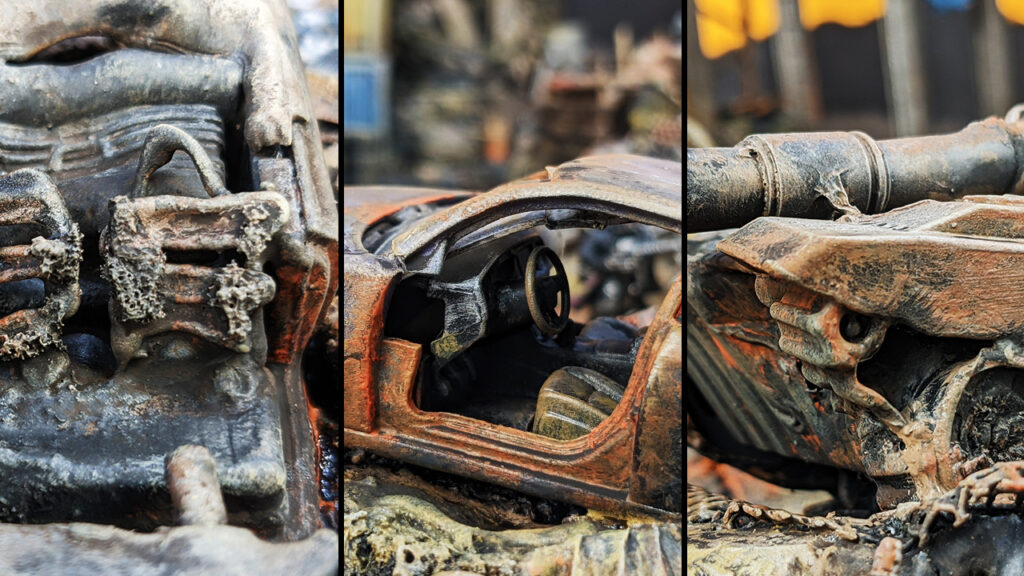The image displays three detailed, close-up photographs of a severely burned and corroded model car. The first photo on the left appears to show what remains of the backseat area, with what look like melted and deformed seat structures, likely plastic, covered in an orange-grey residue. The middle photo provides a more comprehensive side view from the driver's side, with the door conspicuously missing. Inside, you can see a distorted steering wheel, dashboard, and the remnants of two seats, all charred and covered in rust or ash. The background is blurred, possibly to highlight the decayed state of the car. The third photo, on the right, is the most ambiguous but seems to focus on interior components, perhaps near the engine area or another indiscernible part of the car, wrapped in rusty, moldy, and ash-covered debris. The vehicle's remnants have an overwhelming orange, grey, and black color palette and hint at an artistic setup, suggesting that the model might be a toy designed to look like a wrecked, burned-out vehicle.